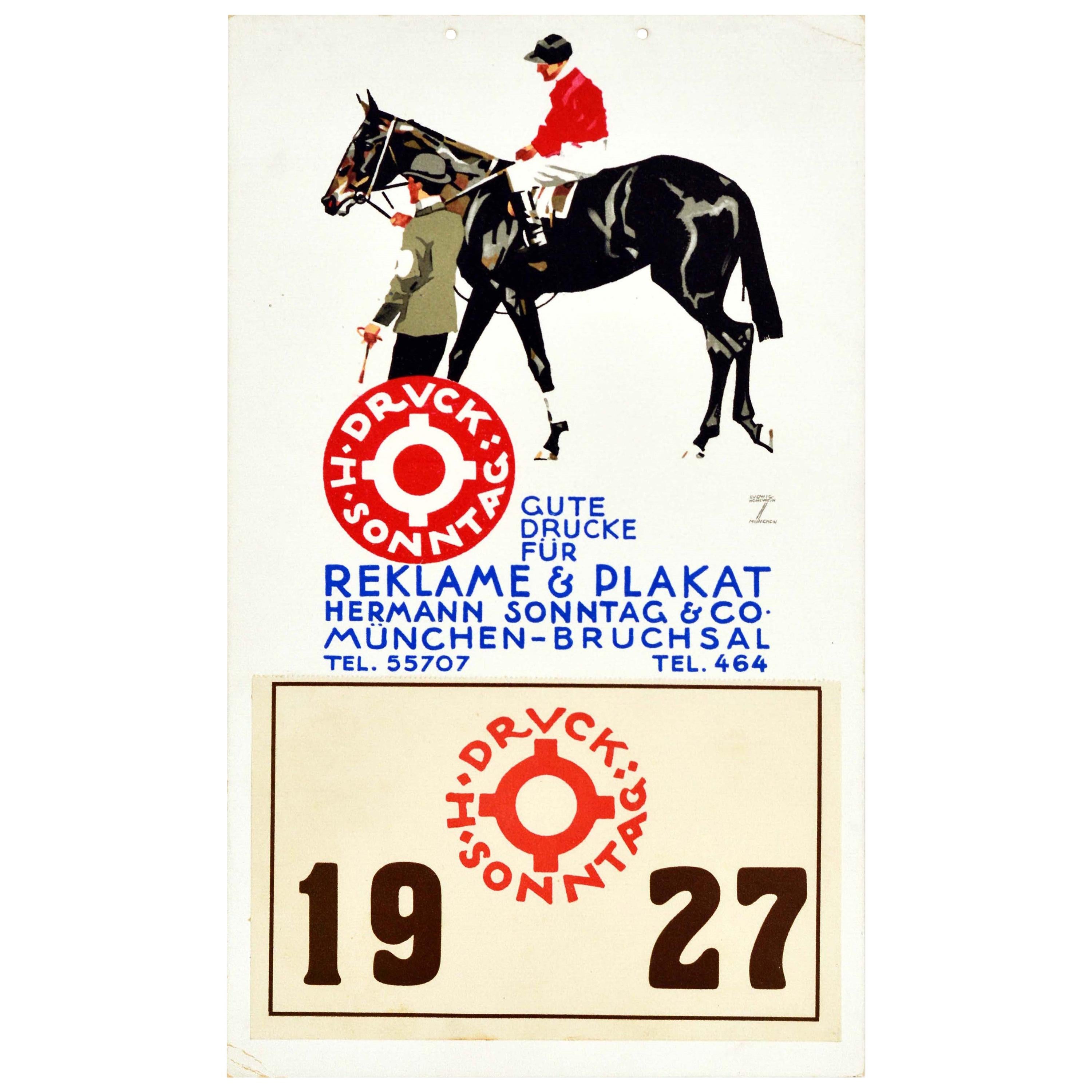This image appears to be a vintage advertisement poster likely related to a horse race, dated 1927. The background is white, and the top section features a detailed drawing of a dark horse in profile, ridden by a jockey. The jockey is dressed in a red jacket, white pants, boots, and a cap. Beside the horse, a man guides it on foot; he is attired in a green jacket, black pants, and wears a top hat. The man appears to be holding an object in his hand, although it is indistinct.

In the center of the poster, there is blue lettering in a foreign language that seems to be German, and also a circular logo with a red cross-like design. Below this text is a tan rectangle where the year "1927" is displayed prominently in brown. The poster also includes several telephone numbers, both five-digit and three-digit, along with additional blue text that is unreadable due to the foreign script. Overall, the dominant colors of the poster are red, green, blue, and black.